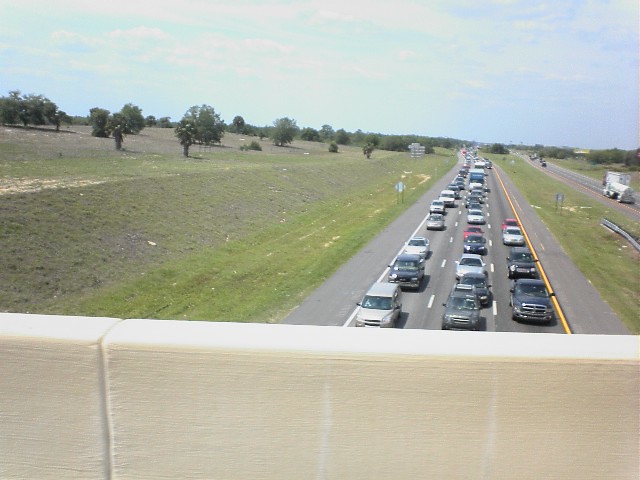The image depicts a daytime traffic jam on a three-lane highway, captured from an overpass or bridge, as evidenced by the railing visible at the bottom of the frame. The congested lanes are filled with a variety of vehicles, including sedans, SUVs, and trucks, all moving in the same direction with no clear end to the backup. The highway is bordered by grassy areas and scattered trees, suggesting a rural or semi-rural setting. In the distance, open land is discernible. The sky overhead is mostly clear with a few scattered clouds. Notably, the far right lane seems to have slightly less traffic than the middle and left lanes. The grass on the left side of the highway is neatly trimmed and extends up a gentle hill dotted with trees. The scene also includes visible street signs and a metal guardrail within the median on the right. The photo, likely taken in the mid-2000s, is of adequate quality, providing a clear view of the traffic conditions and surrounding environment.